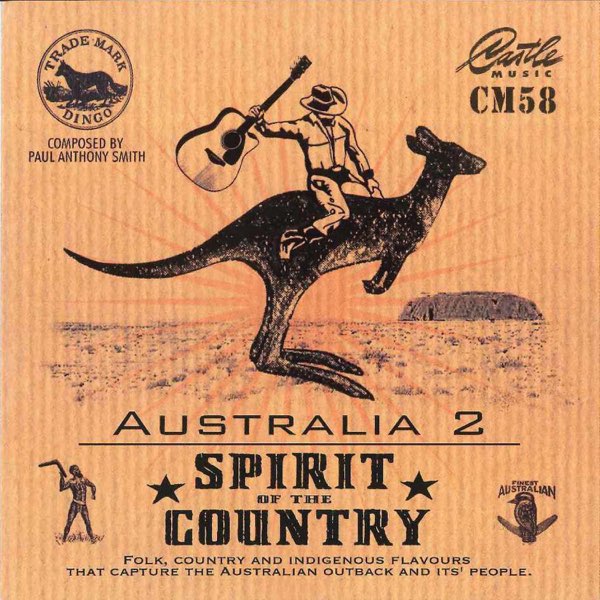The photograph features an album cover predominantly in orange hues with a corrugated, cardboard-like texture. In the top left corner, a circle encloses an image of a dingo looking left, with black text curving around it that reads "Trademark Dingo." Surrounding this is more black text stating "Composed by Paul Anthony Smith." Over on the top right, "Castle Music CM58" is written, with "Castle" in cursive and "CM58" in larger, uppercase letters.

Dominating the center of the image is a cowboy, his face obscured by a tilted hat, riding a kangaroo and holding a guitar triumphantly above his head. Below this vibrant scene are the words "Australia 2," followed by a horizontal line flanked by stars. Under the line is the phrase "Spirit of the Country," in capital letters.

On the lower left side of the cover, a mostly naked man is depicted in mid-motion, about to throw a boomerang. Meanwhile, the right side features the text "Finest Australian" next to an illustrated bird and a tree. Completing the description at the bottom, in black text, are the words "Folk, Country, and Indigenous flavors that capture the Australian outback and its people." This album art vividly encapsulates the essence of Australian culture and the outback spirit through its striking imagery and design.